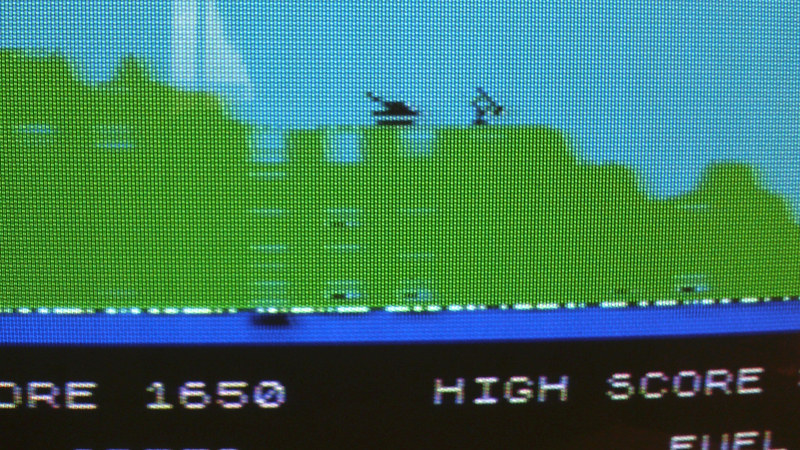This image is a still shot from an old-school video game, likely played on a PC or a TV in the early days of gaming. The image has a slightly blurry look to it, characteristic of early digital graphics. At the very bottom of the screen, there's a black section displaying the text "ORE" followed by "1650," which likely represents the player's score and a high score indicator. Above this, a blue area depicted as water features a small, indistinct black object that might be a boat. The next level up shows a richly green landscape with additional bodies of water on the opposite side. In the background, both a sailboat and another type of boat are faintly visible, adding depth to the scene. The image evokes a nostalgic charm, reminiscent of classic adventure or simulation games from the past.